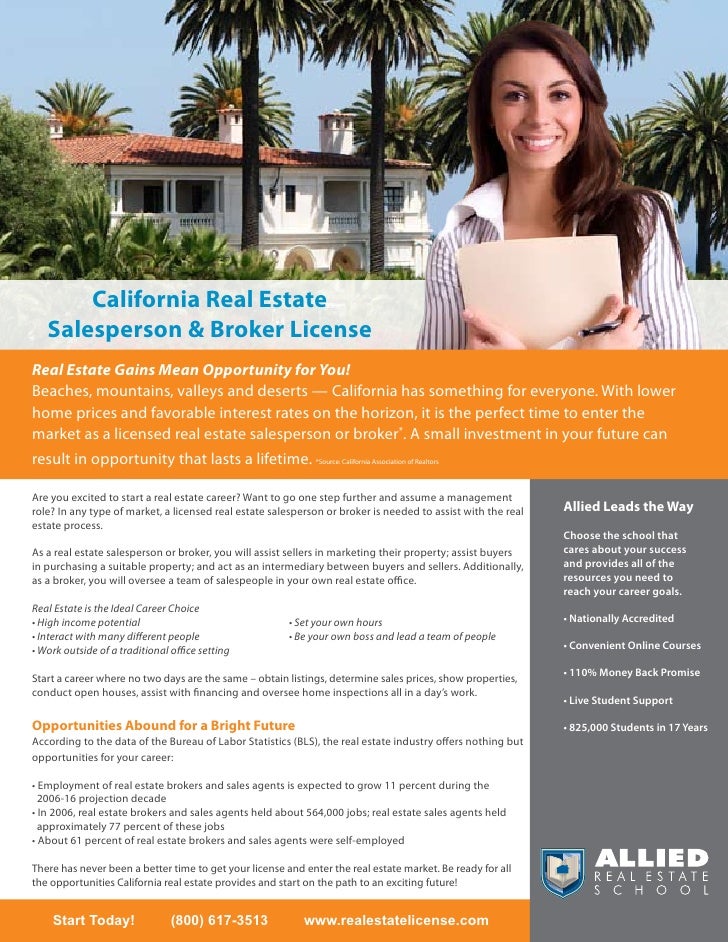This is an advertisement for Allied Real Estate School prominently featuring a grand white mansion with a red roof situated amidst palm trees, suggesting a Southern California setting. The vibrant scene is brightened by the early evening light casting shadows on the mansion. Below this eye-catching image is a smiling young woman on the right, holding a piece of paper, likely representing success in obtaining a California Real Estate Salesperson and Broker License.

On the left of the woman, bold blue letters declare, "California Real Estate Salesperson and Broker License." Below this, an orange box with white text enthusiastically states, "Real estate gains mean opportunity for you!" Additionally, a gray box to the right asserts, "Allied leads the way," providing further information about the institution. On the left, a tan box with black letters explains the benefits and opportunities of a career in real estate or management, underscoring why becoming a real estate agent is a prudent choice. The ad also highlights the allure of California's diverse geography, including beaches, mountains, valleys, and deserts, and emphasizes the present market advantages with lower home prices and favorable interest rates. At the bottom of the ad, contact details are provided, encouraging prospective students to start today by calling 800-617-3513 or visiting www.realestatelicense.com.